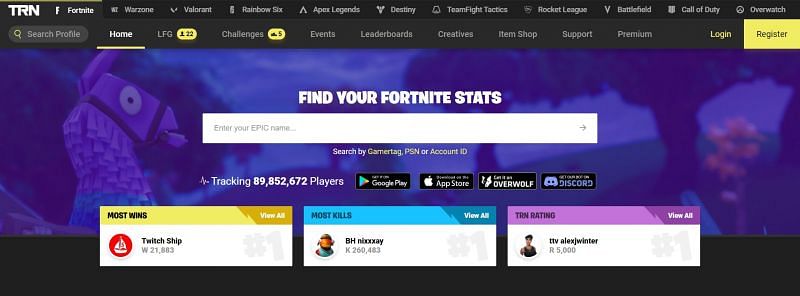The image shows a sleek, black-themed website designed for gaming statistics and profiles with a focus on Fortnite. In the top-left corner, the site features the logo "TRN" accompanied by the word "Fortnite." Adjacent to this, there's a prominent search bar labeled "Search Profile." 

The top navigation bar displays tabs for various popular games: Warzone, Valorant, Rampage 6, Apex Legends, Destiny, Team Fight Tactics, Rocket League, Battlefield, Call of Duty, and Overwatch. Below this main navigation, secondary tabs include Home, LFG (Looking for Group), Challenge, Event, Leaderboards, Creatives, Item Shop, Support, and Premium options. A green "Login" button and a prominently highlighted green "Register" button are also located at the top.

Centrally located on the page, bold text invites users to "Find your Fortnite stats," accompanied by a search field that instructs "Enter your Epic name, search by gametag, PSN, or account ID." Just below this, a subtitle notes the impressive number of players tracked by the platform: 89,852,772.

Further down, the website highlights user achievements and statistics, featuring three specific sections:
- On the bottom left, with a yellow background, it showcases the "Most Winning Twitch," noting a total of 21,703 wins.
- Next, with a blue background, it displays "Most Kills," attributed to user "bhnikze" with an astounding 260,483 kills.
- Lastly, with a purple background, it features the "TRN Rating," showcasing "ttvalexjwinter" with a rating of 5,000.

The bottom section also includes patterns referring to integration/services like Cookieplay, Appstore, Overwolf, and Discord, enhancing the website’s community connectivity and feature set.